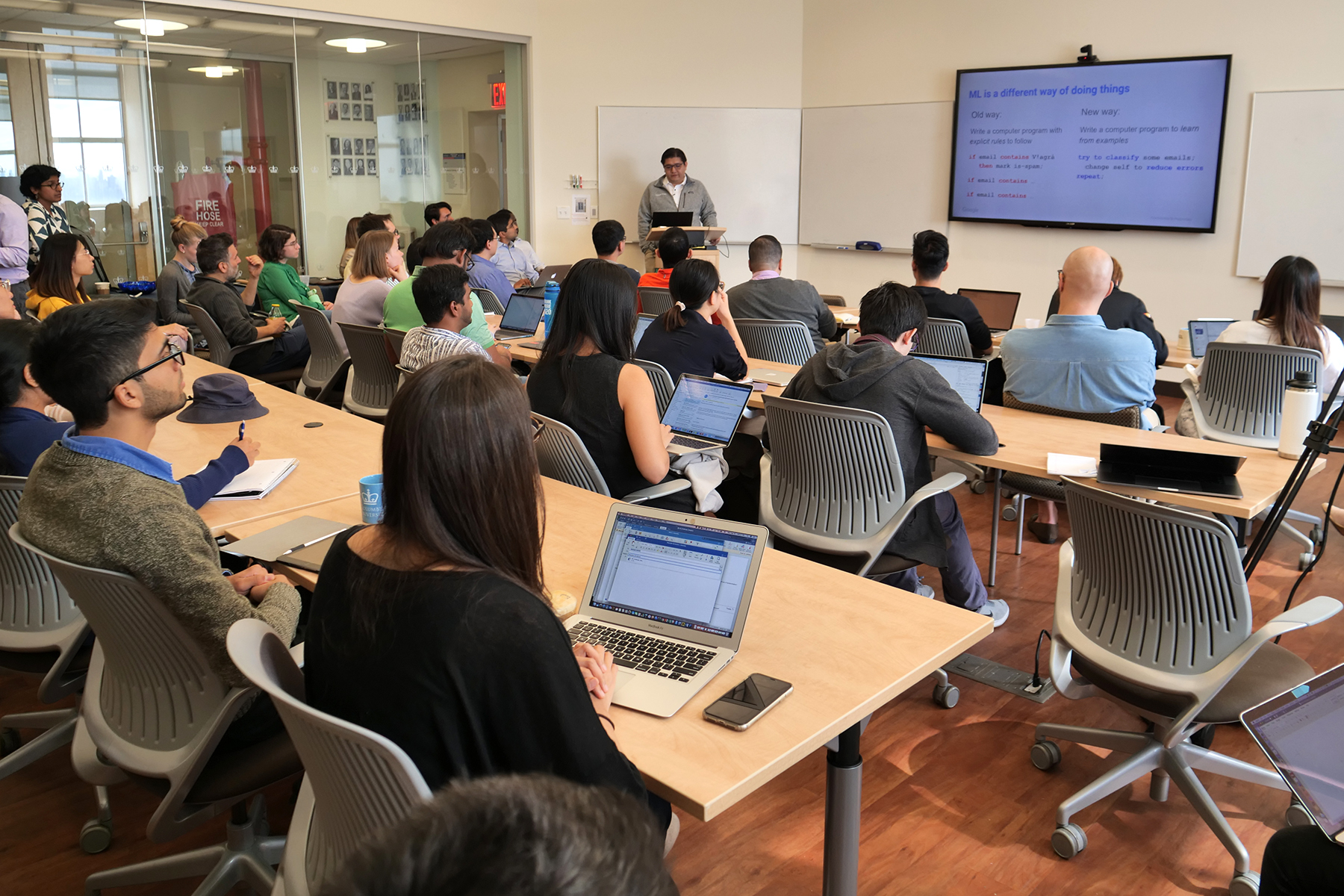This photograph captures an indoor scene of a diverse, multi-age group of students attending a seminar or lecture, likely at a college or university. The space is organized with three rows of long wooden tables, occupied by students seated in light gray office chairs. Most of the students are using laptops, though some are taking notes with paper and pencil, and a few are on their phones. From our vantage point at the back of the room, we see the students' backs as they face the front of the room.

At the front, a woman stands at a podium, giving a speech with her laptop open in front of her. She is positioned to the left of the room's front wall, which is beige and features three whiteboards. Between the whiteboards, a large projection screen displays a slide that reads, "ML is a different way of doing things," comparing the "old way" with the "new way." 

The room's floor is a mid-tone wood, and on the upper left, there's a glass wall revealing signage that says "fire hose." The instructor, a man with dark hair, glasses, and a gray sweatshirt, captures the attention of the room as he delivers his lecture. The setting exudes a focused and engaged learning environment.